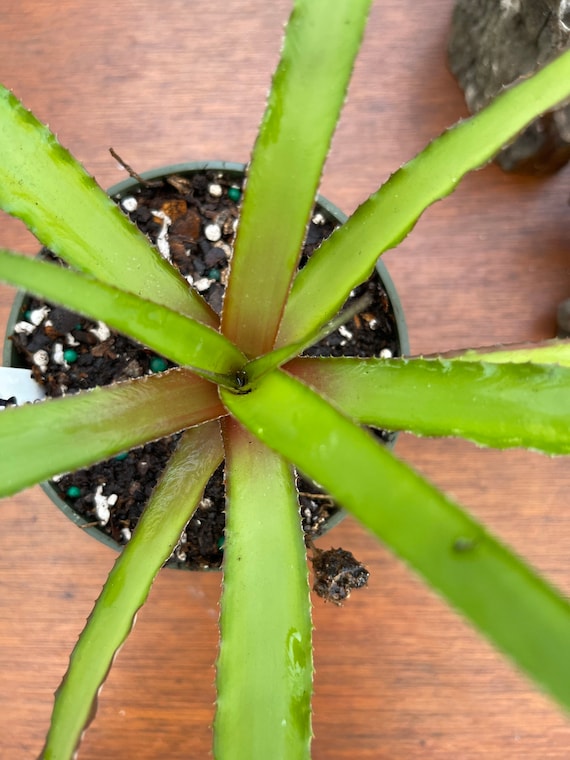This aerial view image showcases a young, healthy aloe vera plant with approximately ten to eleven long, slender, smooth green leaves. The plant appears vibrant and well-nurtured, with leaves that have a slight reddish-brown tint near the center. Planted in a black plastic pot, the aloe vera is surrounded by a potting mix that includes wood chips, vermilion, and white fertilizer chunks. Additional elements like small red stones and blue circular balls, potentially plant food, are also visible in the soil mixture. The pot is placed on what looks like a wooden table, indicated by the visible wood grain surface beneath it. Overall, the scene depicts a thriving aloe vera plant in an organized and aesthetically pleasing environment.